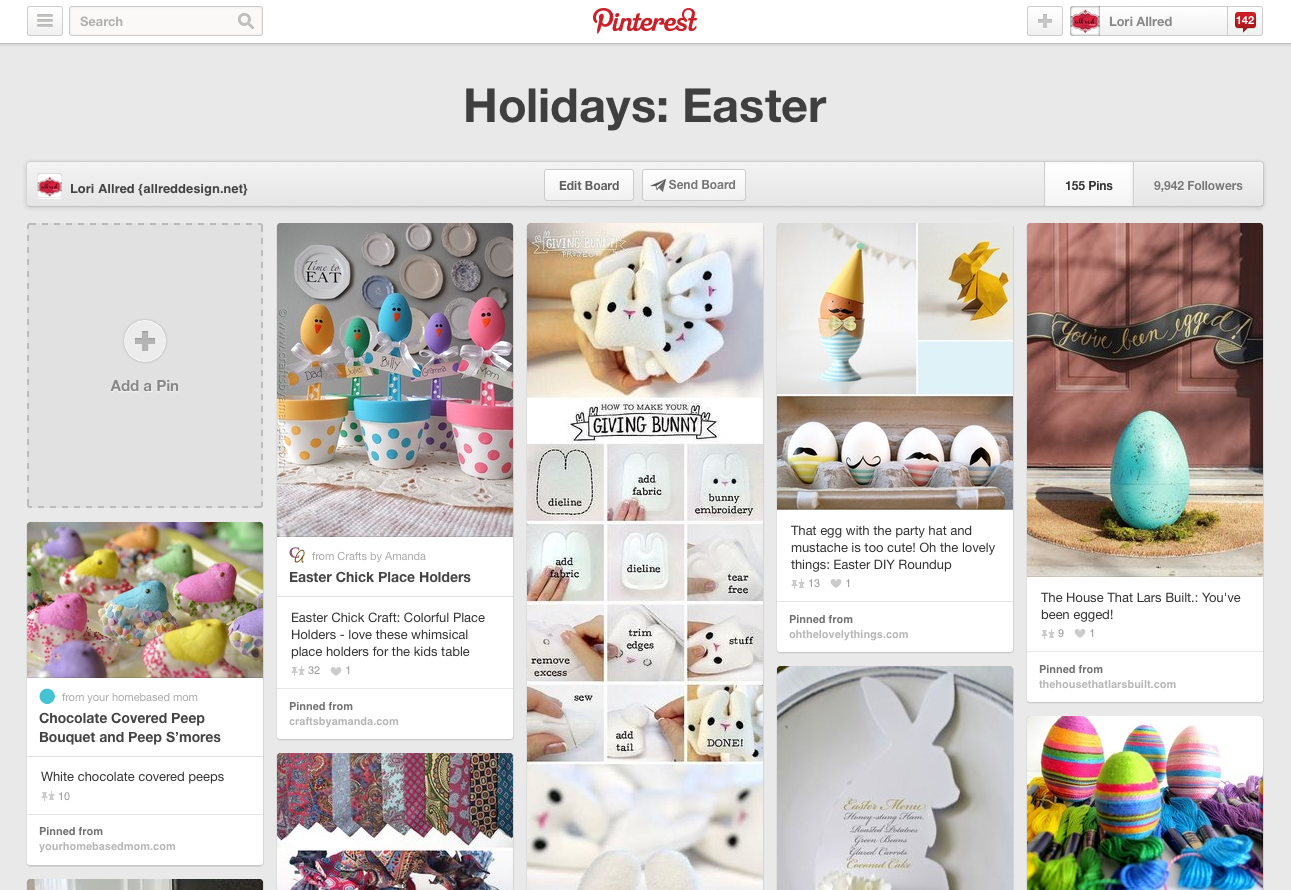The website of Pinterest has a distinct layout with a clean white background. In the upper left-hand corner, there's a white square containing three gray horizontal lines, which appears to be a menu icon. Adjacent to this is an off-white rectangular search bar, outlined in gray, and containing a light gray magnifying glass icon.

At the center top, the Pinterest logo is prominently displayed in red, rendered in a cursive script. On the right side, there is a small gray square featuring a light gray plus sign, probably for adding new pins.

Next to it is another gray-outlined square with white and red colors inside. Alongside this is a light gray search box with the text "Lost Abroad" written inside it. Below the header, the site transitions to a gray background.

In the middle section, under the Pinterest logo, bold black text reads "Holidays... Easter." Below this, there is a section for adding new pins with the label "Add a Pin" in gray, surrounded by various existing pins. The pins include captions such as "Easter Chick Placeholders," "Easter Chick Craft," "Colorful Placeholders," "Love These Ones," "Group Placeholders," "Most Kids at the Table," "Chocolate-Covered Peep Bouquet," "Peep S'mores with Chocolate-Covered Peeps," and "That House That Lars Built." One particular pin of interest reads "You've Been Egged" and is accompanied by an image of a green egg.

This detailed layout description captures the organized and visually engaging interface of Pinterest.